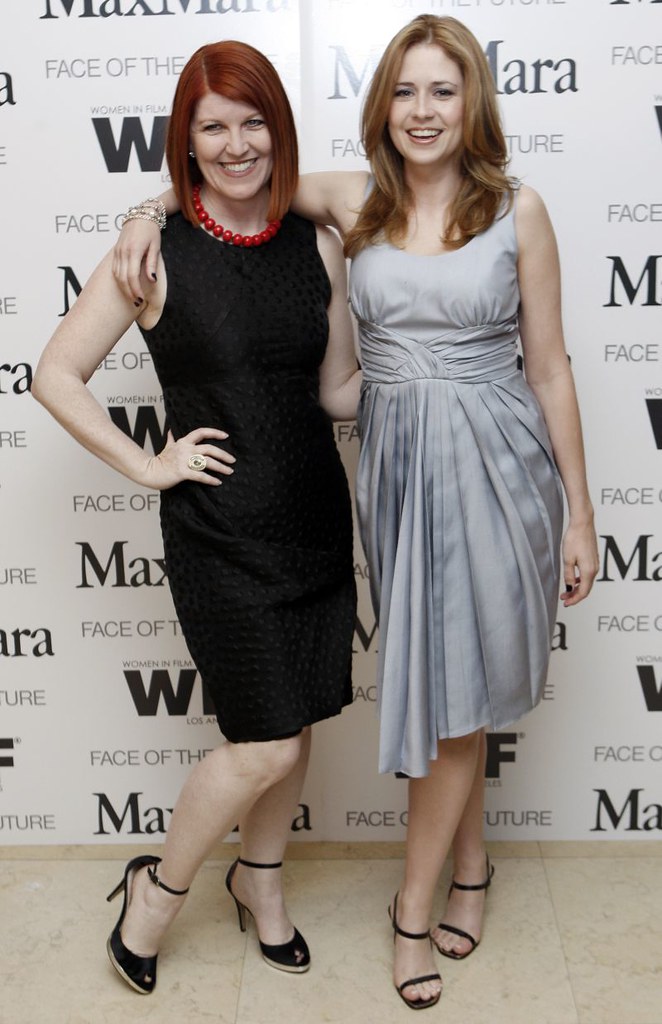The image features two actresses from the TV show "The Office" standing and posing for the picture against a white background patterned with the words "Max Mara Face of the Future." On the left is a white woman with shoulder-length straight brown hair, wearing a black sleeveless dress paired with black high heels and a large red beaded necklace. She has her arm around the shoulder of the other woman. On the right, there is another white woman, known as Pam from the show, with straight red hair. She wears a sleeveless silver dress, black high heels, and has one hand placed on the center of the other woman's back while the other rests on her hip. Both are smiling directly at the camera, standing on a light beige tiled floor.